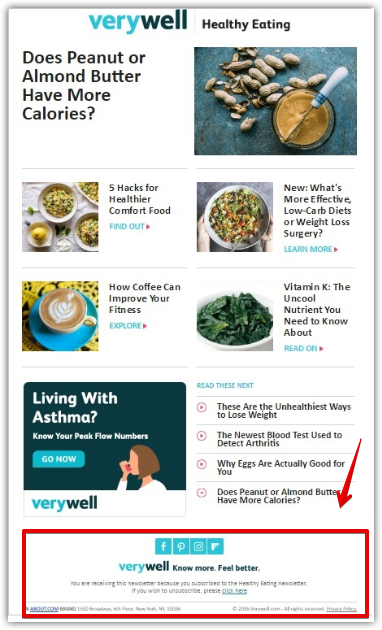This is a detailed screenshot captured from the "VeryWell" website, showcasing various blog post titles and sections on a white background. The site name, "VeryWell," is stylized with "Very" in turquoise and "Well" in dark blue, although it does not feature a logo. 

At the top, a main heading poses the question: "Does peanut or almond butter have more calories?" Below this are various content highlights: 

- A graphic of peanut butter next to the text "Five Hacks for Healthier Comfort Food."
- A new article titled "What's More Effective: Low Carb Diets or Weight Loss Surgery?" accompanied by a "Learn More" link.
- An informative post titled "How Coffee Can Improve Your Fitness" with an accompanying coffee image and an "Explore" button.
- A section on "Vitamin K: The Uncool Nutrient You Need to Know About" with a "Read On" prompt.
- A health segment labeled "Living with Asthma: Know Your Peak Flow Numbers," featuring a "Go Now" button for more details.

Additionally, the screenshot includes a red arrow pointing to a section marked with social media icons, indicating integration with various social media platforms.